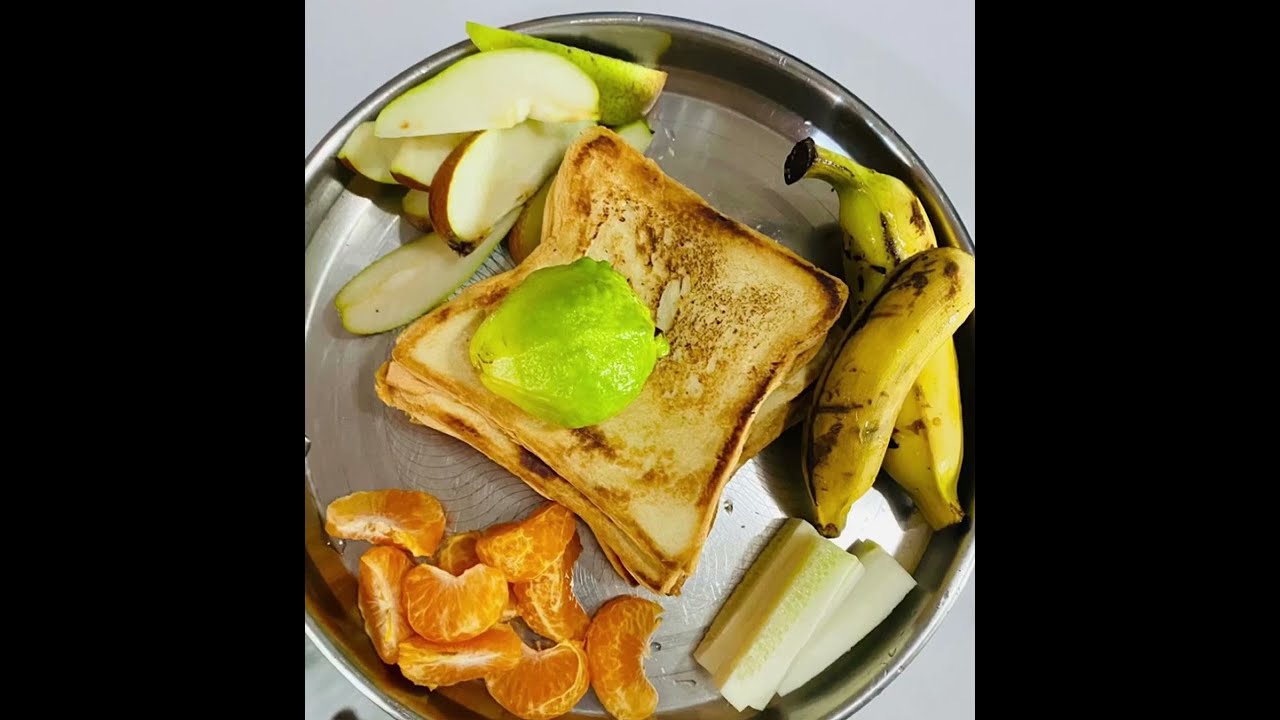This is an overhead photograph taken from above a round, shiny silver metal plate, showcasing a variety of food items laid out for what appears to be breakfast. At the center of the plate, there are two pieces of toast, with a bright green avocado half resting on top. The toast may have some kind of spread between the slices. Surrounding the toast are different fruits and some additional items: to the top left, there are slices of green apple revealing their white flesh inside; to the bottom left, there are segments of peeled tangerines, providing a burst of vibrant orange color; to the right of the toast, there are two baby bananas with yellow and slightly green skins; and on the bottom right, there are slices of off-white cheese or possibly cucumber sticks with a light green hue. Additionally, there are some sliced carrots on the top left part of the plate, near the apples. The entire arrangement is placed on a light blue surface with two vertical black strips flanking the image on both sides, reminiscent of a photo commonly seen on Instagram.